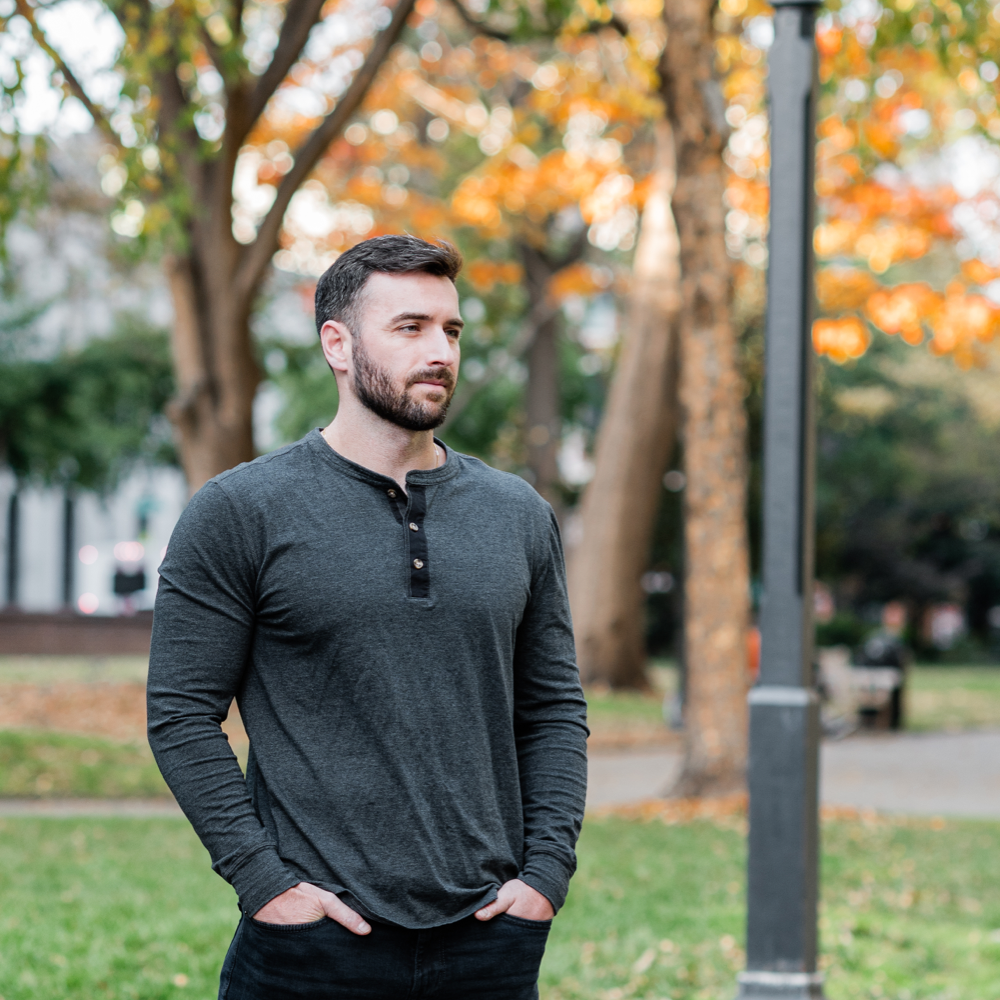This photograph captures a thoughtful, middle-aged Caucasian man with dark hair, a dark beard, and dark eyes, dressed in a dark gray long-sleeved shirt with black trim and black pants. He stands with his hands in his pockets, gazing off to the right side of the frame. Behind him, a park-like setting stretches out with a mix of green and orange-hued fall foliage, hinting at the autumn season. A light post is nearby, and a light gray walking trail meanders through the green grass. The background is slightly blurred, showcasing various trees with light brown trunks and vibrant leaves. The scene suggests a crisp fall day, partly cloudy and void of other people, highlighting the man's pensive demeanor.